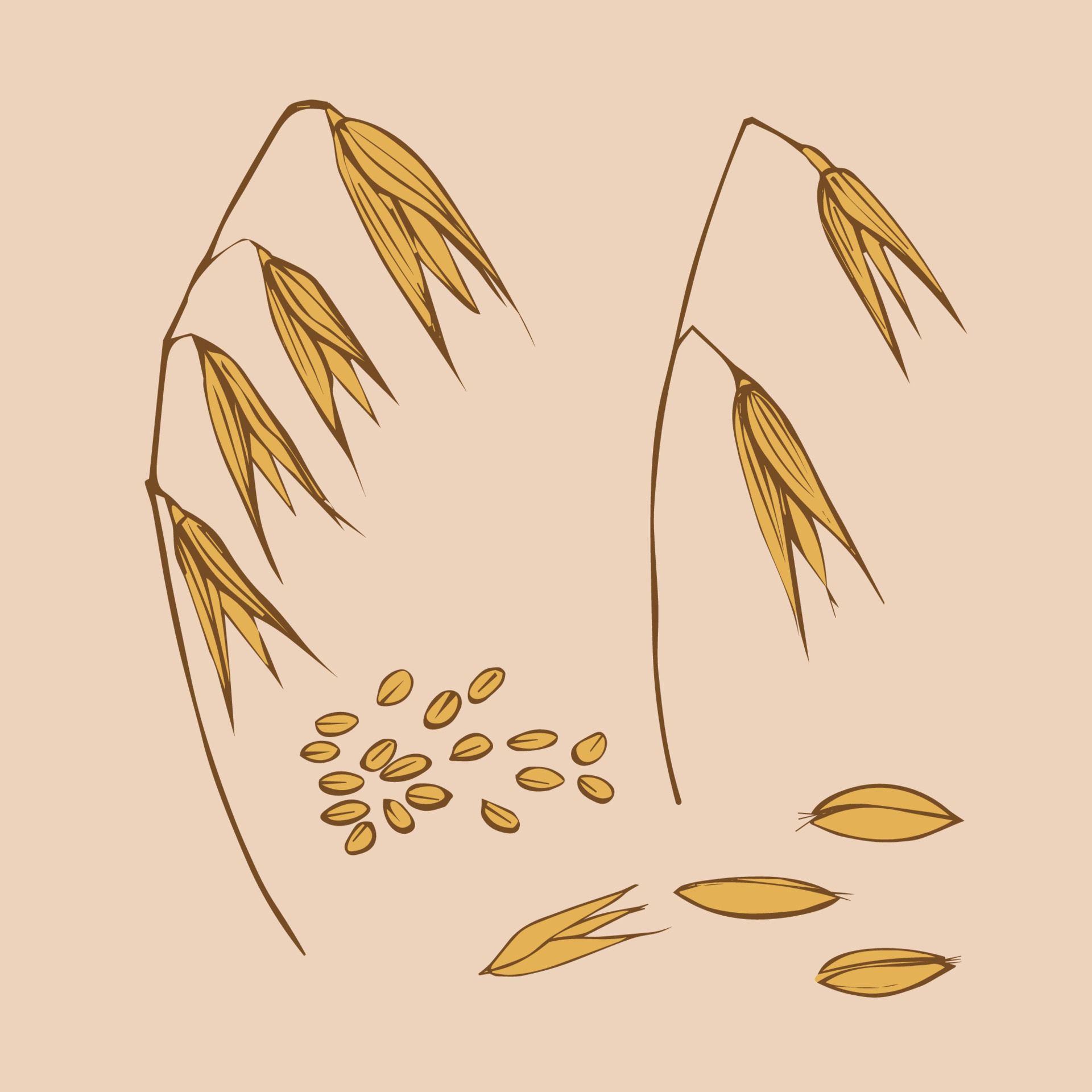The image depicts a detailed drawing of two dried wheat stalks against a flat matte pink background. The wheat stalks, rendered in tan with dark outlines, lean slightly to the side. The stalk on the left features four pods of leaves, while the stalk on the right has two pods, both displaying a droopy appearance as if they are wilting. Scattered around the base of the stalks lie numerous kernels and detached pods, estimated to be around 12 or 13 in total. These elements are positioned primarily in the bottom left and right corners of the image, adding a sense of decay and earthiness to the scene. The overall composition, with its cartoonish style and softened hues, captures the somber beauty of dried, aged flora.